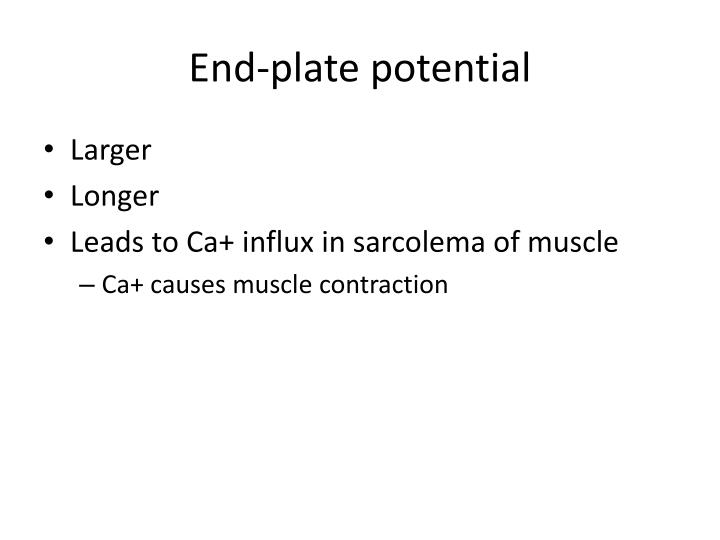The image features a simple and straightforward text-based slide, likely part of a larger slideshow presentation. The background is plain white, and the title at the top center reads "End-Plate Potential" with a capitalized "E" in "End." The text is black and possibly in Arial font, with the title slightly larger (around 14 point font), compared to the content (around 12 point font for bullet points and 10 point font for the sub-bullet). Below the title are three bullet points. The first bullet point reads "Larger," the second bullet point reads "Longer," and the third bullet point states "Leads to Ca²⁺ influx in sarcolemma of muscle." Following the third bullet point, a sub-bullet indicated by a dash notes that "Ca²⁺ causes muscle contraction." All of the text is neatly formatted, displaying essential information concisely, likely intended for educational purposes.